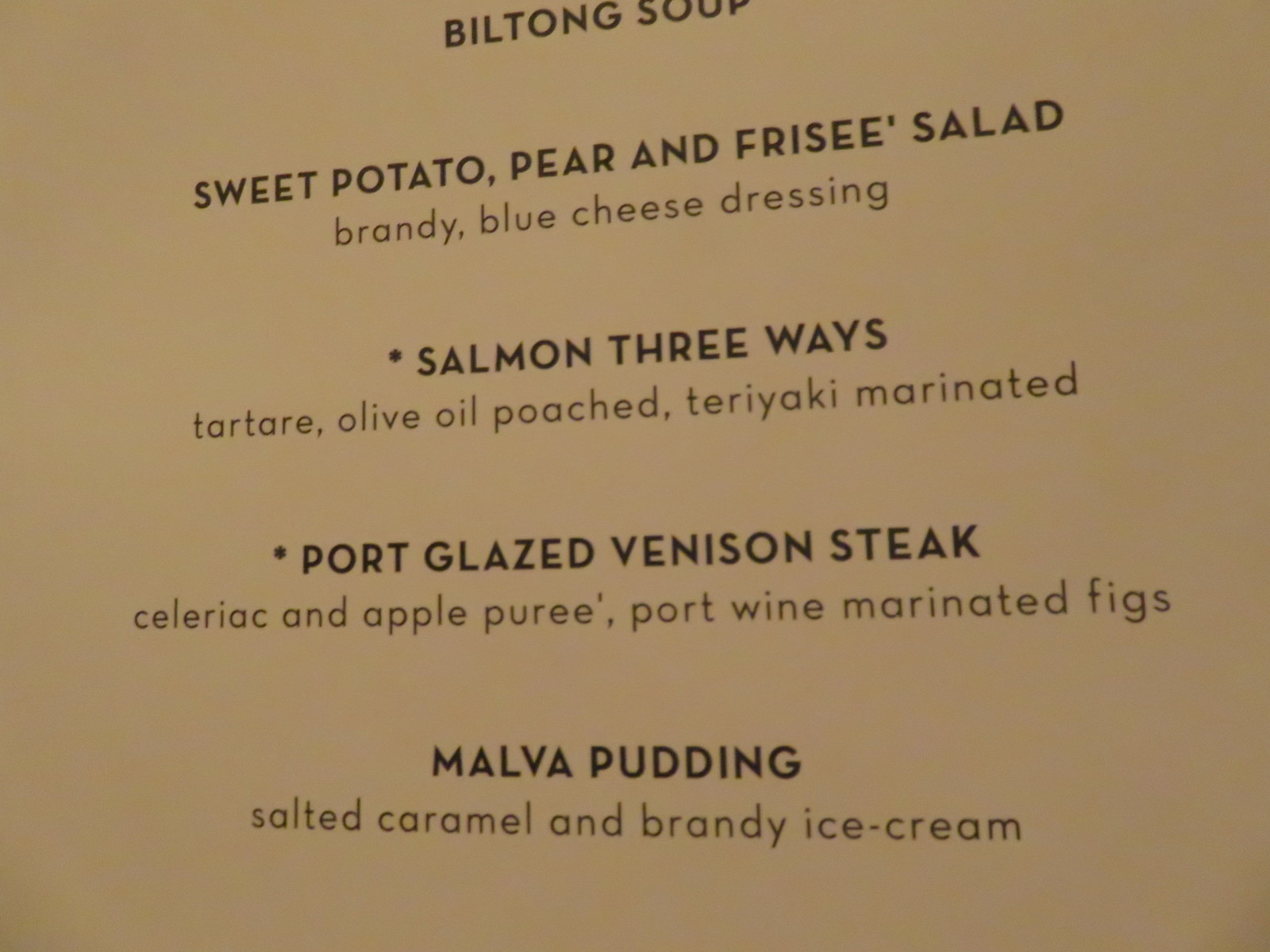The image features a sophisticated and elegantly designed menu with a dark tan background and black text, center-justified for a streamlined, refined aesthetic. At the top, in bold black lettering, the menu title reads "Biltong Soup." Following beneath, the first dish is "Sweet Potato, Pear, and Frisee Salad" with intricately described ingredients including brandy and blue cheese dressing. The second entree, marked with an asterisk, is "Salmon Three Ways," prepared in three distinct styles: tartare, olive oil poached, and teriyaki marinated. Next, "Pork Glazed Venison Steak" is highlighted, accompanied by celeriac and apple puree, and port wine marinated figs, offering a rich, complex flavor profile. The dessert section lists "Malva Pudding" served with salted caramel and brandy ice cream. The menu layout allows ample space between each item, enhancing readability and emphasizing each dish's unique components, contributing to an overall impression of luxury and culinary finesse.